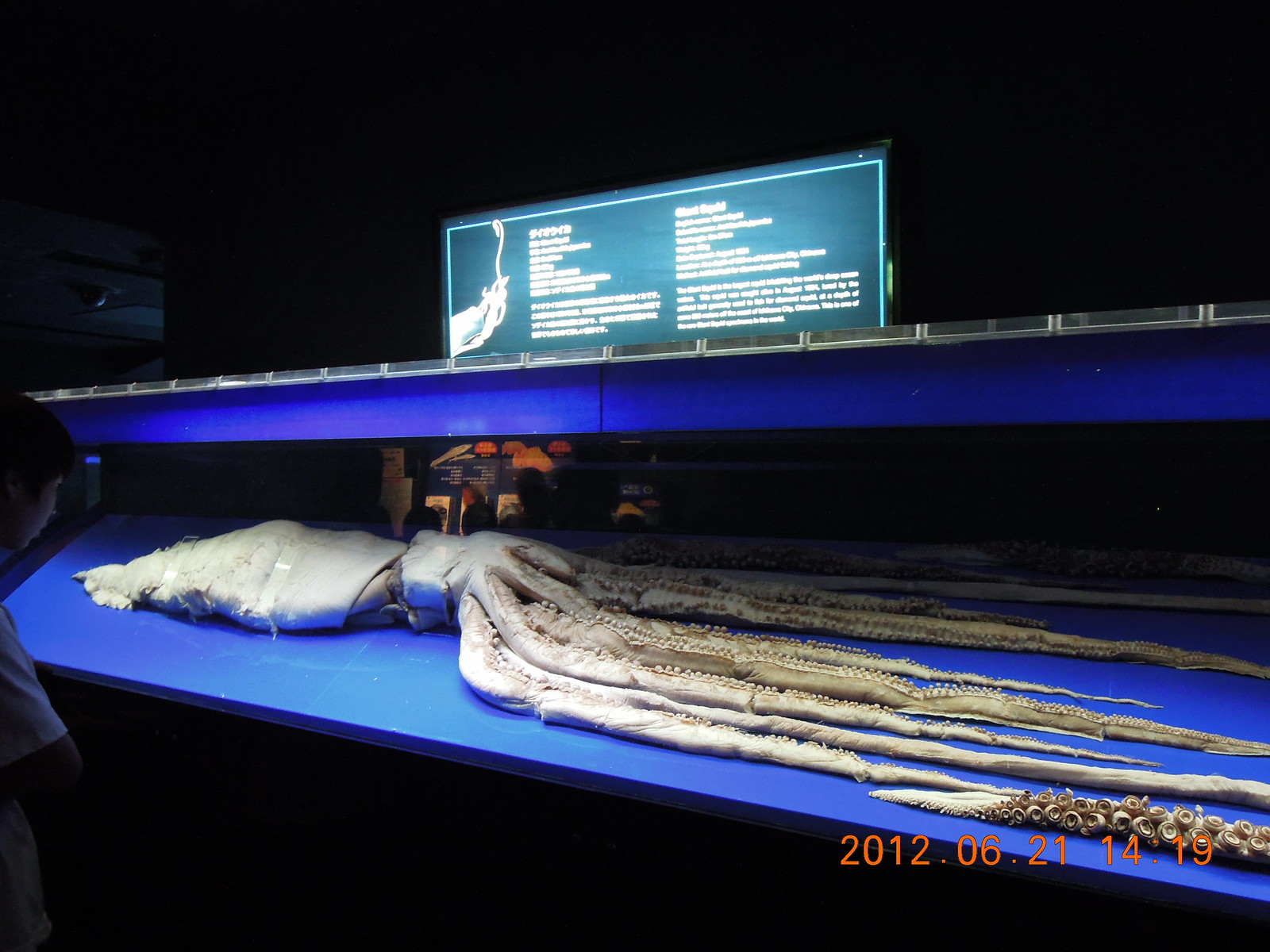This night-time photograph showcases an enormous squid, potentially an octopus, displayed across two medium blue platforms arranged in two levels. The platforms, likely serving as tables or staging areas, stand against a pitch-black backdrop. The squid, an off-white color, dominates the image with its head positioned around the top left, around 40% from the left edge, stretching its numerous tentacles diagonally down to the bottom right, occupying about 10% of the photo's height. Measuring without scale but clearly extensive in length, the cephalopod appears lifeless, possibly removed from a tank and placed for display or study. Above the platforms is a green sign adorned with white text, obscured and unreadable. Additionally, the bottom right corner of the image is marked with the date 2012-06-21, suggesting the photo's capture date.